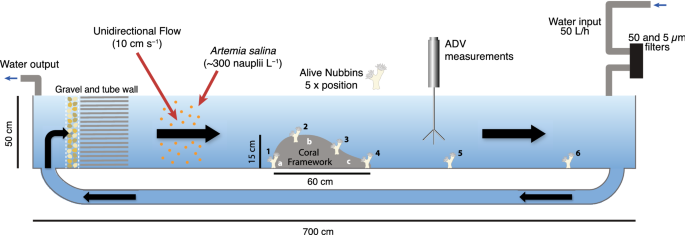This image is a detailed infographic illustrating the osmosis process, focusing on water input and output through various stages. The central structure resembles a see-through blue rectangle, akin to a bathtub, measuring 50 centimeters in height and spanning 700 centimeters in length. The overall design is primarily light blue with black arrows indicating the water flow direction, accompanied by gray elements for contrast.

The process begins with water input, marked by text and arrows. The water enters the structure and travels through a tube located under the rectangle. It then passes through a gravel and tube well, followed by a section labeled "coral framework." Subsequent phases include passing an ADV measurement area and a section marked "unidirectional flow." The process also features specific details such as "Artemia salina" and "alive nubbins."

Each stage is accompanied by text boxes that provide descriptions and measurements, ensuring clarity and aiding in following the flow of water through the system. The arrangement of the elements is horizontal, enhancing readability and emphasizing the step-by-step progression of the osmosis process.